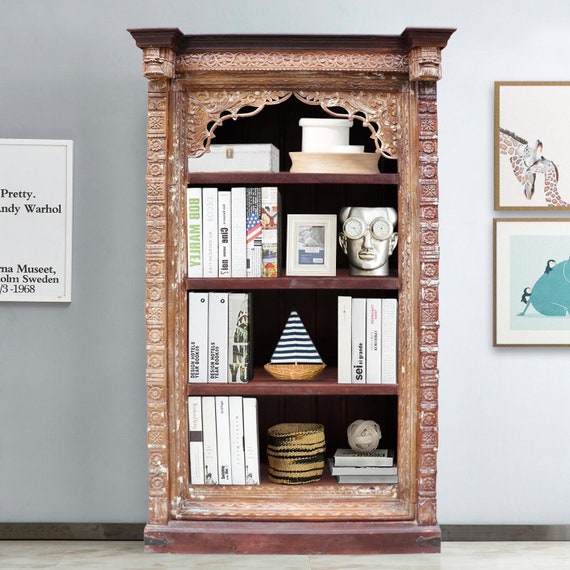The image features an ornately detailed wooden bookshelf set against a light gray wall with a brown trim at the base. The floor, faintly visible at the bottom of the image, is tan or beige. The bookshelf is large, reaching nearly from the bottom to the top of the image, and is made of wood, showcasing intricate patterns and carvings around its edges. The base of the bookshelf is a darker, reddish-brown color. 

The bookshelf contains four shelves, each filled with various items:
- The top shelf displays a case and several small decorative objects.
- The third shelf houses a peculiar statue of a head wearing goggles, a picture frame, and a few books.
- On the second shelf, centrally positioned, is a small sailboat, flanked by three books on the left and four on the right. 
- The bottom shelf holds five books to the left, a basket in the center, and three books stacked horizontally on the right with a small spherical decoration on top.

To the right of the bookshelf on the wall are two paintings: the upper painting depicts two giraffes, while the lower one features a corporate art style image that partially shows an elephant. Partially visible text on the wall hints at information related to Andy Warhol and potentially a museum exhibit, with fragments like "pretty," "must sect," "Stockholm, Sweden," and "1968."